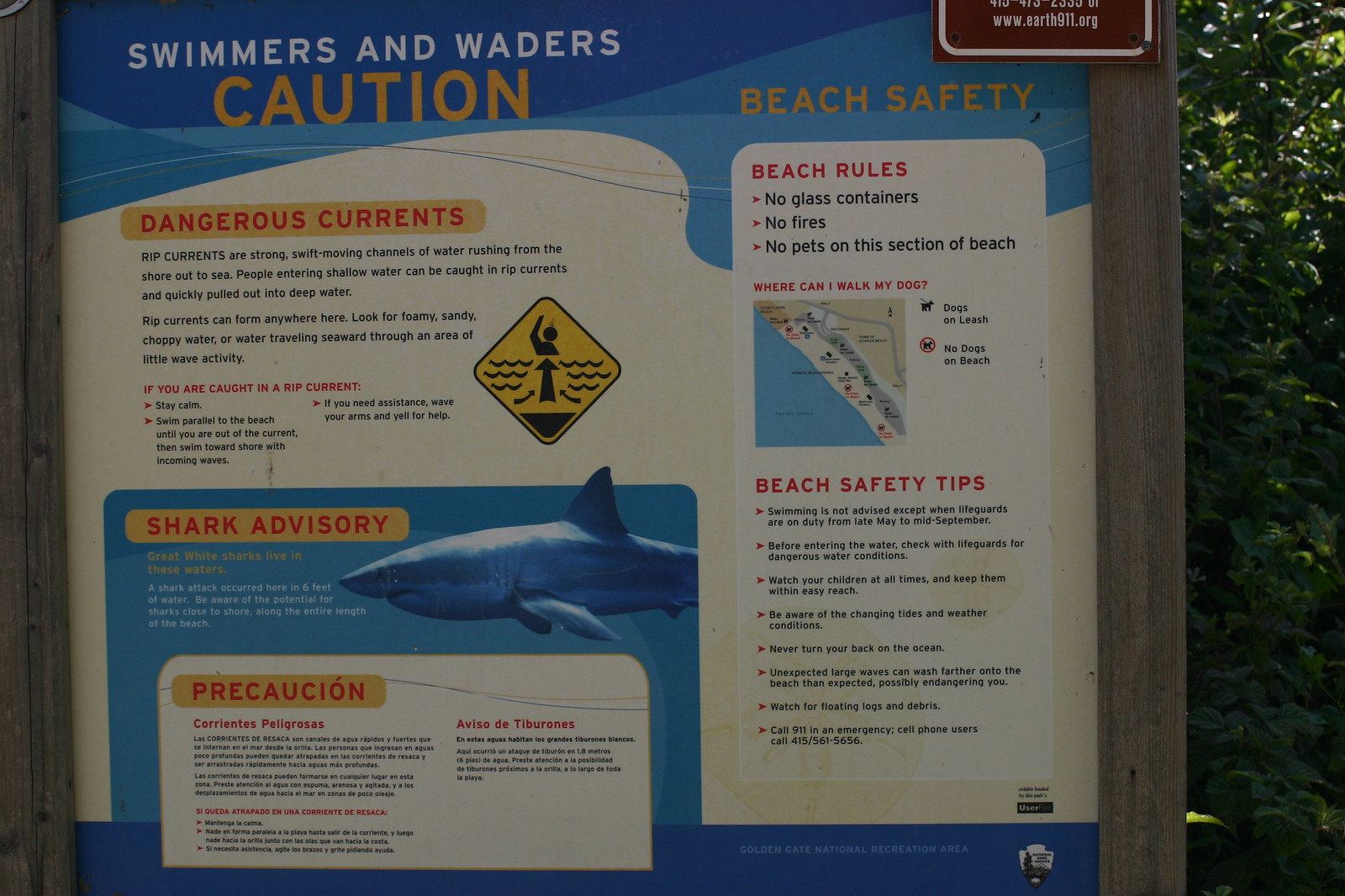The image shows a detailed outdoor wooden-framed sign positioned at a beach, with bushes visible in the background. The sign is filled with various safety warnings and rules, highlighted with bold headers in blue, white, yellow, and red. At the top, it prominently warns swimmers and waders of dangerous rip currents, explaining the nature of these currents and advising that if caught, one should stay calm and swim parallel to the shore, or wave their arms and yell for help if assistance is needed. 

Directly below this section, the sign also features a shark advisory with an image of a great white shark, cautioning that these sharks inhabit the waters and offering safety precautions in both English and Spanish. 

On the right side of the sign, there is an array of beach safety tips that include not swimming unless lifeguards are on duty (from late May to mid-September), always checking with lifeguards for dangerous water conditions, vigilantly watching children, and being aware of changing tides and weather. Additional tips include not turning your back on the ocean to avoid unexpected large waves and avoiding floating logs and debris.

The sign also lays out beach rules: no glass containers, no fires, and no pets allowed on this section of the beach. There is a color-coded map displaying designated areas where dogs can be walked on a leash and where they are not permitted on the beach. Emergency contact information, such as calling 911 or, for cell phone users, dialing 415-561-5656, is also provided for quick access in case of emergencies.